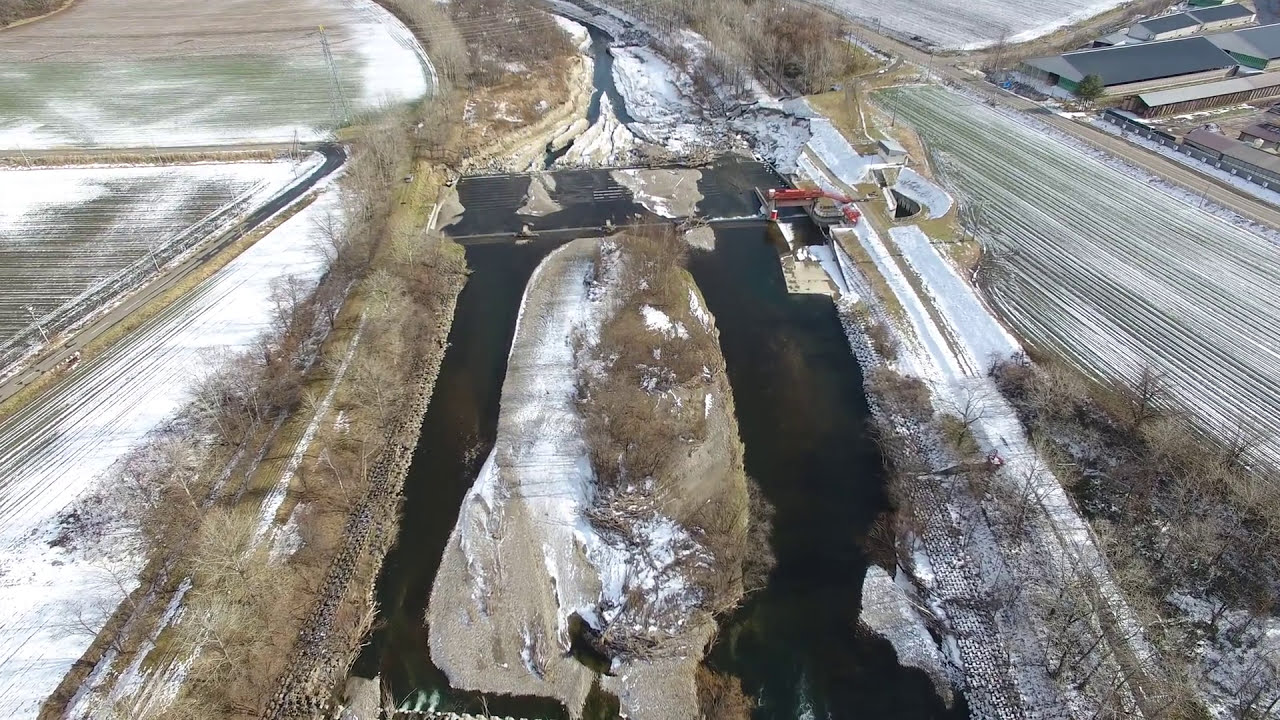This aerial photograph depicts a winter scene centered on a water treatment plant. At the top middle of the image, a snow-dusted stream branches into a Y-shape before feeding into an inlet surrounded by pipes. This inlet connects to a large pool or pond featuring a small island adorned with trees. The pond is bordered by a road and a snowy field, likely used for growing wheat or corn. The landscape is covered in a light layer of snow, indicating winter, with trees stripped of their leaves. To the right of the field lies a larger barn with a black roof, flanked by two smaller buildings. The entirety of the scene captures the essence of a rural farmland area with natural colors of brown, green, white, gray, and black. The photograph also shows some low-lying buildings, towers, and scattered areas of dirt and grass, emphasizing the agricultural setting.